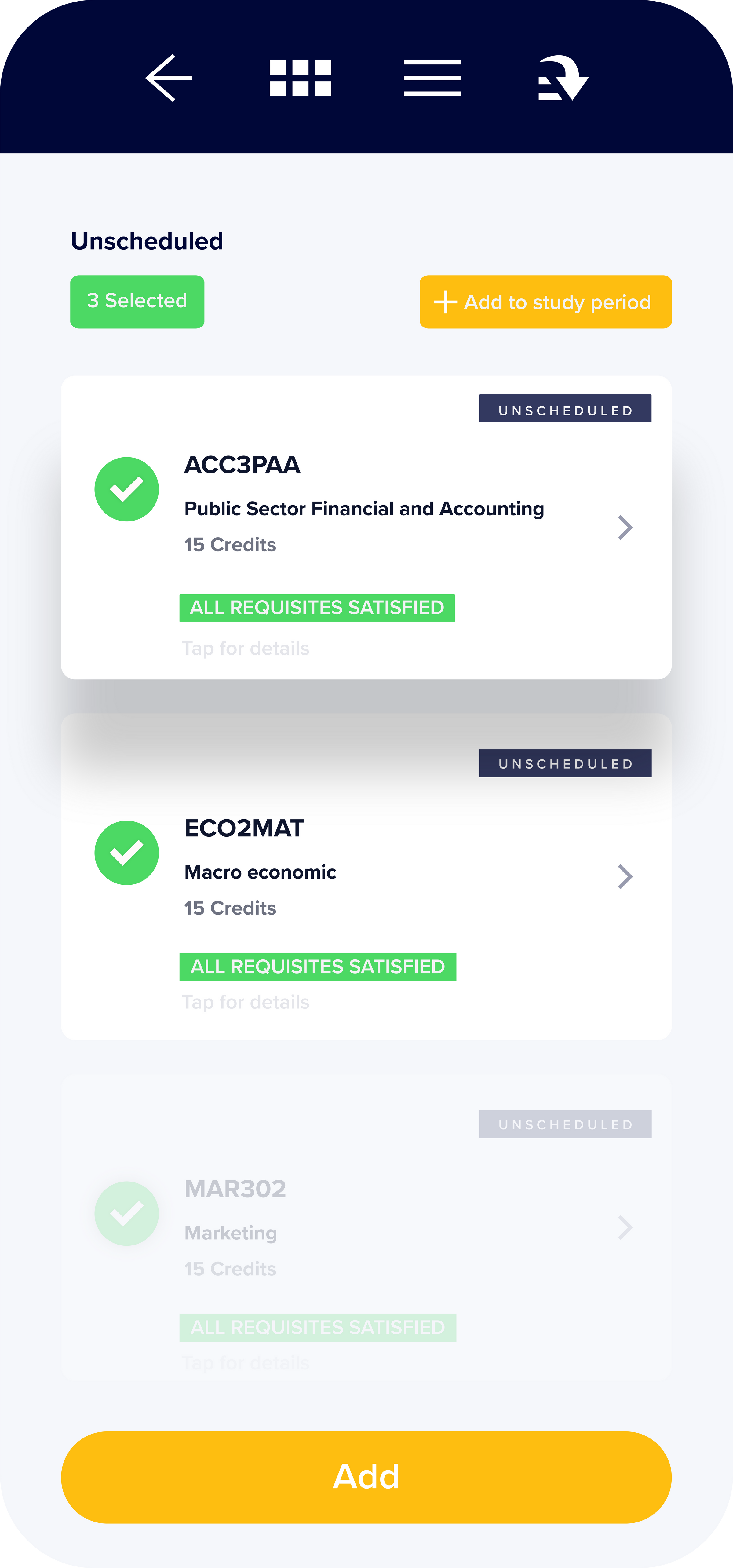This screenshot depicts a mobile app's settings screen, specifically focusing on an academic schedule interface. The interface features a sleek black background with white icons. At the top, there is a black menu bar that includes a left-facing white arrow, followed by two rows of three small white squares, likely an icon representing the app's home or main menu. To the right of the squares, there is a trio of horizontal lines, a common symbol for additional menu options. On the far right, there is a downward-pointing arrow indicating a dropdown menu or additional options.

Beneath this menu bar, the background shifts to light gray, with dark blue and dark gray text. The header at the very top reads "Unscheduled," indicating this section covers courses that have not yet been integrated into the user's timetable. Below the header, there are two prominent boxes: a green box with white text stating "3 selected" and a yellow box with white text that says "Add to Study Period."

The schedule visible in this section lists three academic courses, each detailed with course codes and information. The first course, clearly visible, is labeled "AC3PAA Public Sector, Financial and Accounting," worth 15 credits, with all requisites satisfied. As you move down the list, the other two courses begin to fade out, indicating their position further down the list. Each entry includes the course's scheduling status at the top, denoted as "Unscheduled."

At the bottom of the screen, beneath the list of courses, there is a button labeled "Add," which allows the user to integrate the selected courses into their study period or timetable. This interface seems to facilitate the organization and planning of the user’s academic schedule, showing pertinent details such as credits and prerequisite fulfillment for each course.